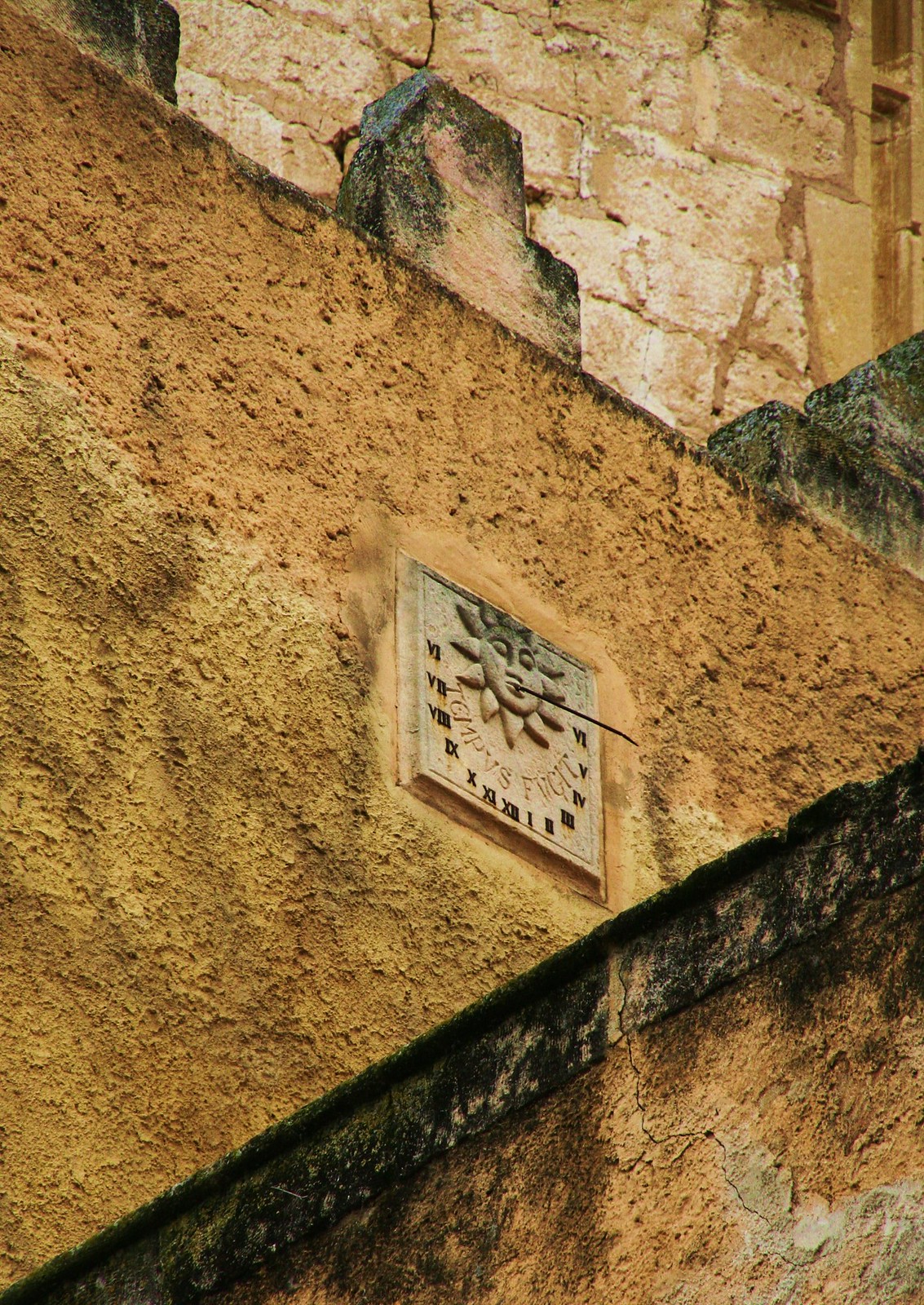This detailed charcoal drawing showcases a weathered city street rendered in a palette of black, tan, beige, and white. Dominating the scene is a concrete sidewalk that has suffered the ravages of time. The wall rising from the sidewalk is aged and crumbling, revealing a patch of broken bricks where the concrete facade has deteriorated. The sidewalk itself is distorted, likely due to a sinkhole, resulting in a dangerous drop of several inches along a sharp edge, an obvious hazard for pedestrians. Adding a unique element to the scene, a square sundial clock is set on the damaged sidewalk, its embossed sun design and a prominently extended second hand accentuating the passage of time and decay in this urban landscape.